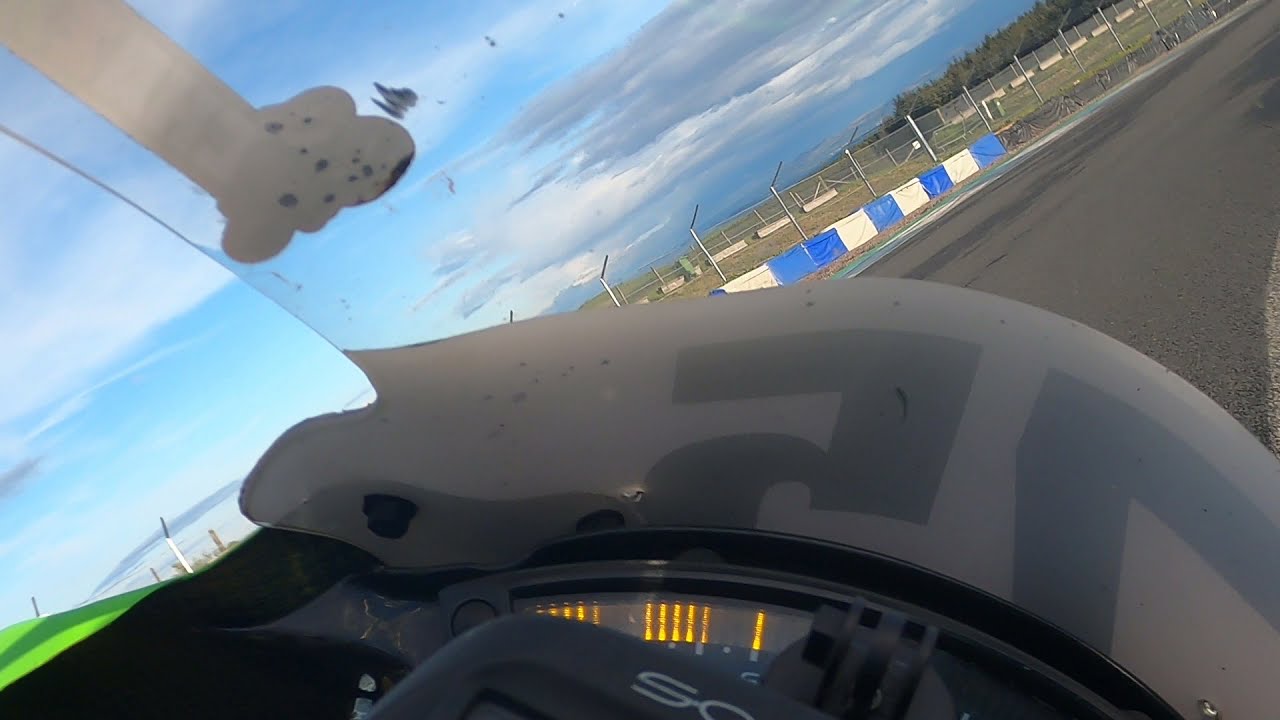The photograph captures a confusing and angled close-up of a motorcycle, seemingly taken by someone mounted on the vehicle. The image is partially obstructed by a rounded grayish bar, likely part of the motorcycle's structure, arching over an odometer or dial. A glass or plexiglass shield with the number 75 is also visible. This shield obstructs a clear view and creates a tilted perspective, suggesting the motorcycle might be navigating a rightward curve but stationary, as indicated by the sharpness of the background details. The scene in the distance features an asphalt track bordered by fences, with green grass, trees, and a road curving to the right. The sky above is blue with clouds, hinting at either early evening or a clear daytime setting. A blue and white siding runs along the fence, possibly indicating a practice field or similar area. Overall, the image captures a blend of motion and stillness, with the motorcycle's structure dominating the foreground and a fenced-off track under a partly cloudy sky in the background.